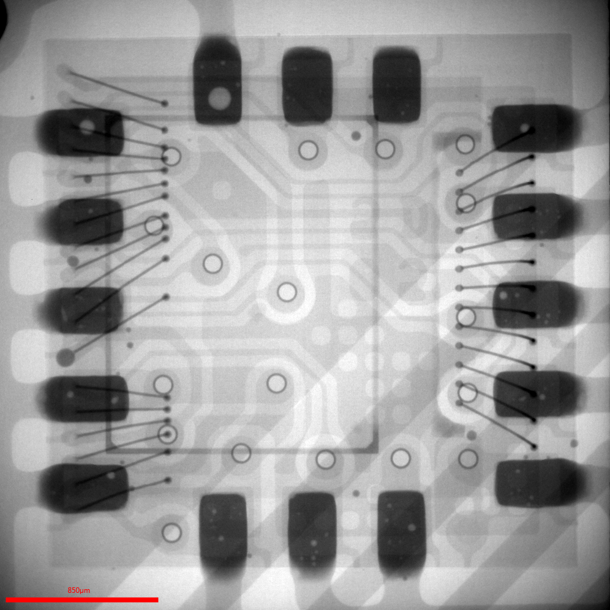The photograph appears to be a highly zoomed-in, microscopic close-up of a circuit board, displaying intricate, light gray and white circuitry patterns against a white background. The circuit board is characterized by a series of connected lines and dots, with several black rectangles arranged along the border, specifically three at the top, three at the bottom, and five on each side, forming a symmetrical pattern. Black lines radiate from the left and right sides, adding to the complexity of the image. At the bottom left corner, there's a small red horizontal line beneath the number "850," which likely indicates a scale of 850 micrometers. The image has a hazy, pixelated, and slightly blurred quality, reminiscent of an x-ray scan, enhancing its intricate and detailed appearance.